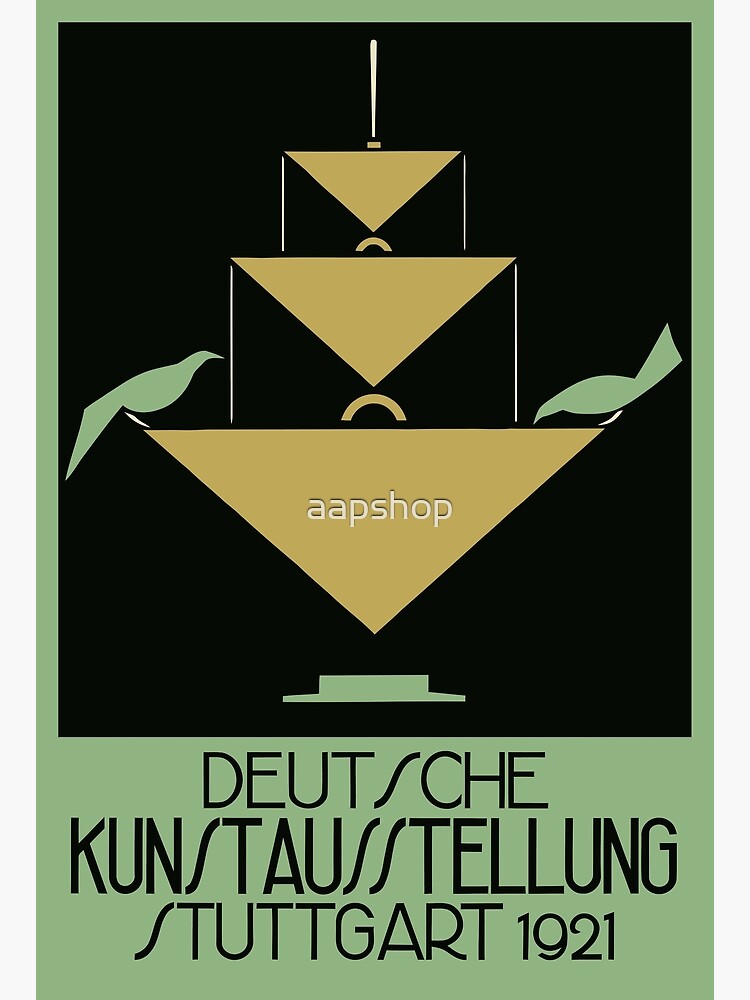This image appears to be an Art Deco styled poster or book cover from 1921, advertising a German art exhibition in Stuttgart. The poster features a deep mint green frame with a wide band at the bottom. This band contains large black italicized text that reads "Deutsche Kunstausstellung Stuttgart 1921," some of the 'S's elongated for stylistic effect. Above this is a black rectangle occupying the top two-thirds of the image, within which lies a gold, tiered, triangle-based geometric design representing a three-tiered fountain. At the apex of each triangle, intricate white lines suggest streams of water cascading downward. The top triangle is the smallest, with each tier increasing in size to form the fountain's structure. On either side of the bottom and largest triangle, two green silhouette birds are positioned—one leaning down as if drinking from the fountain, the other with its head bowed. In the middle of the largest triangle is white text that reads "AAP shop," and beneath this, a green saucer-like base complements the design. The overall aesthetic is distinctly 1920s, characterized by its angular lines and bold, limited color palette of deep mint green, black, gold, and white.